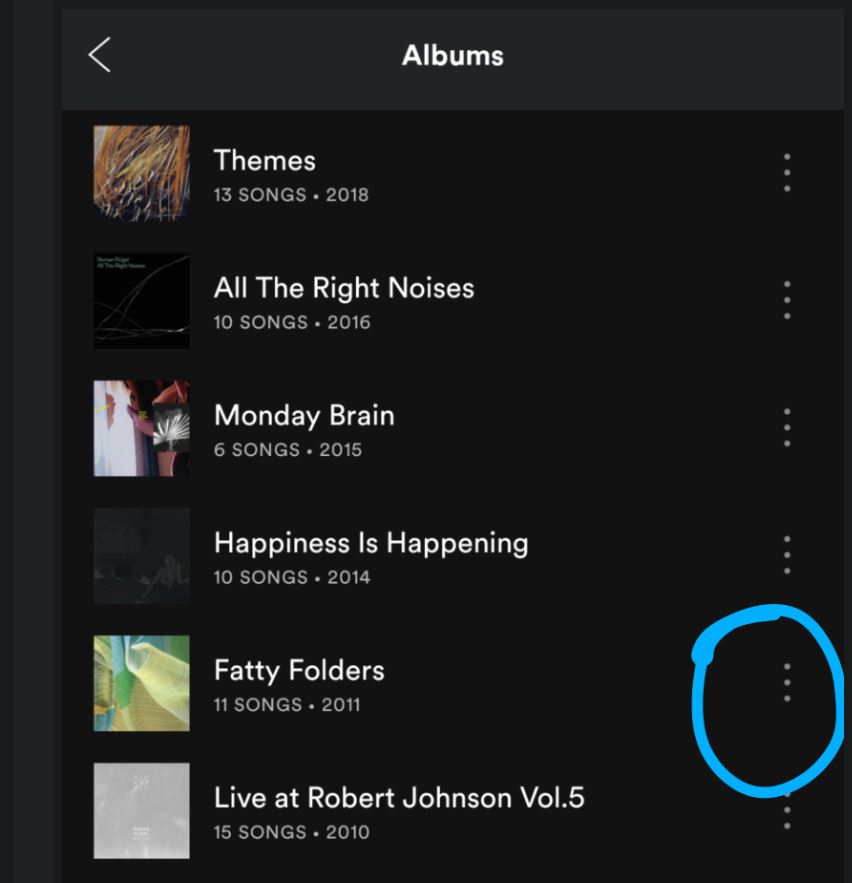This image features a sleek, black background, prominently displaying the word "Albums" at the top in bold, white font. Positioned at the top left corner is a left arrow symbol. Just below the title "Albums," there are six album covers arranged in a visually appealing layout.

1. The first album, titled "Themes," is from 2018 and contains 13 songs.
2. The second album, "All the Right Noises," dates back to 2016 and includes 10 songs.
3. "Monday Brain," the third album, was released in 2015 and comprises 6 songs.
4. The fourth album, "Happiness is Happening," hails from 2014 with a collection of 10 songs.
5. The fifth album, "Fatty Folders," is from 2011 and features 11 songs.
6. The final album, "Live at Robert Johnson Volume 5," was released in 2010 with 15 songs.

Each of these albums is represented by a unique cover, adding visual diversity to the image.